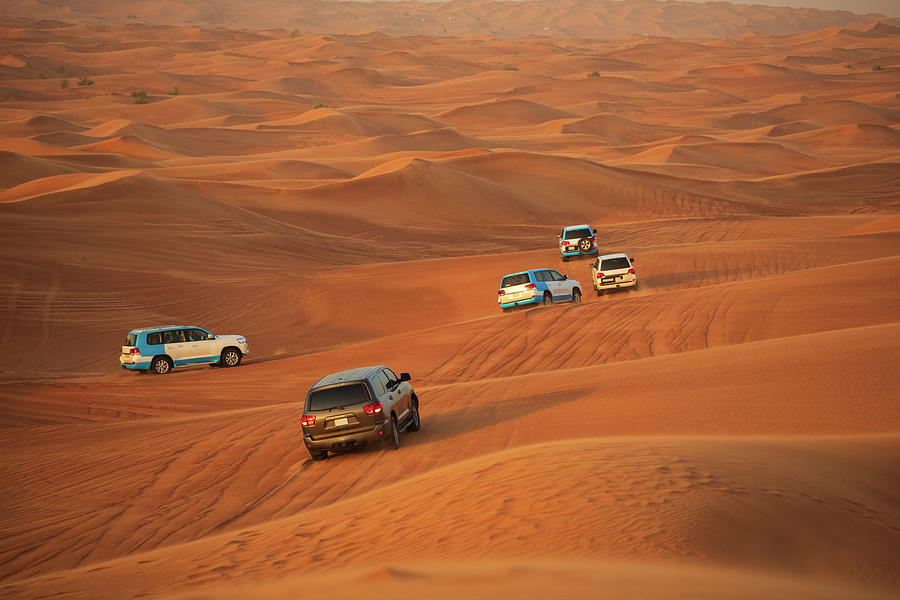The photograph captures five sports utility vehicles traversing a sprawling, hilly desert landscape characterized by dark umber sand interwoven with shades of orange and brown. The undulating terrain is peppered with scattered scrub brushes, adding specks of greenery to the otherwise arid expanse that stretches endlessly into the distance. The desert scenery hints at a Middle Eastern setting, notable for its distinctive light and shadow interplay, creating a somewhat surreal ambiance.

The vehicles are positioned in a line, moving away from the camera, with tracks and dust trailing behind them, highlighting their movement across the sandy hills. The leading vehicle is blue and white, followed in succession by a white one, two more blue and white vehicles, and finally, a darker, brownie-green-gray vehicle approaching from a slightly different angle. Notably, the vehicle furthest from the camera has a spare tire mounted on its rear. All the vehicles are illuminated by daylight, making the details of their exteriors vividly apparent and emphasizing their uniformity in model but slight variations in paint jobs.